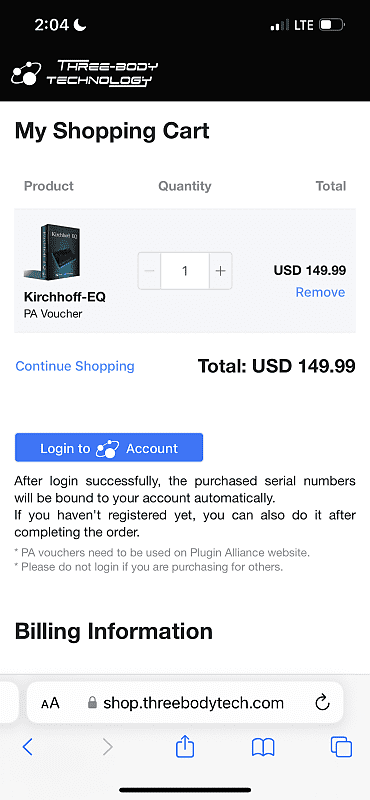A screenshot of the shopping cart area on the website shop3bodytech.com. The website URL appears at the bottom of the image, while the header displays "Shop 3 Body Technology." The section is titled "My Shopping Cart" and includes column headers for "Product," "Quantity," and "Total." The product listed is a "Kerchoff EQ PA Voucher," with a quantity of one and a total price of USD $149.99. Below this, a summary states the "Total: USD $149.99." Instructions at the bottom inform the user to "Login to Account," stating that after a successful login, the purchase serial numbers will be automatically bound to the account. It also mentions that if the user hasn't registered, they can do so after completing the order. A cautionary note advises that PAVE vouchers need to be used on the Plugin Alliance website and warns not to log in if purchasing for others.